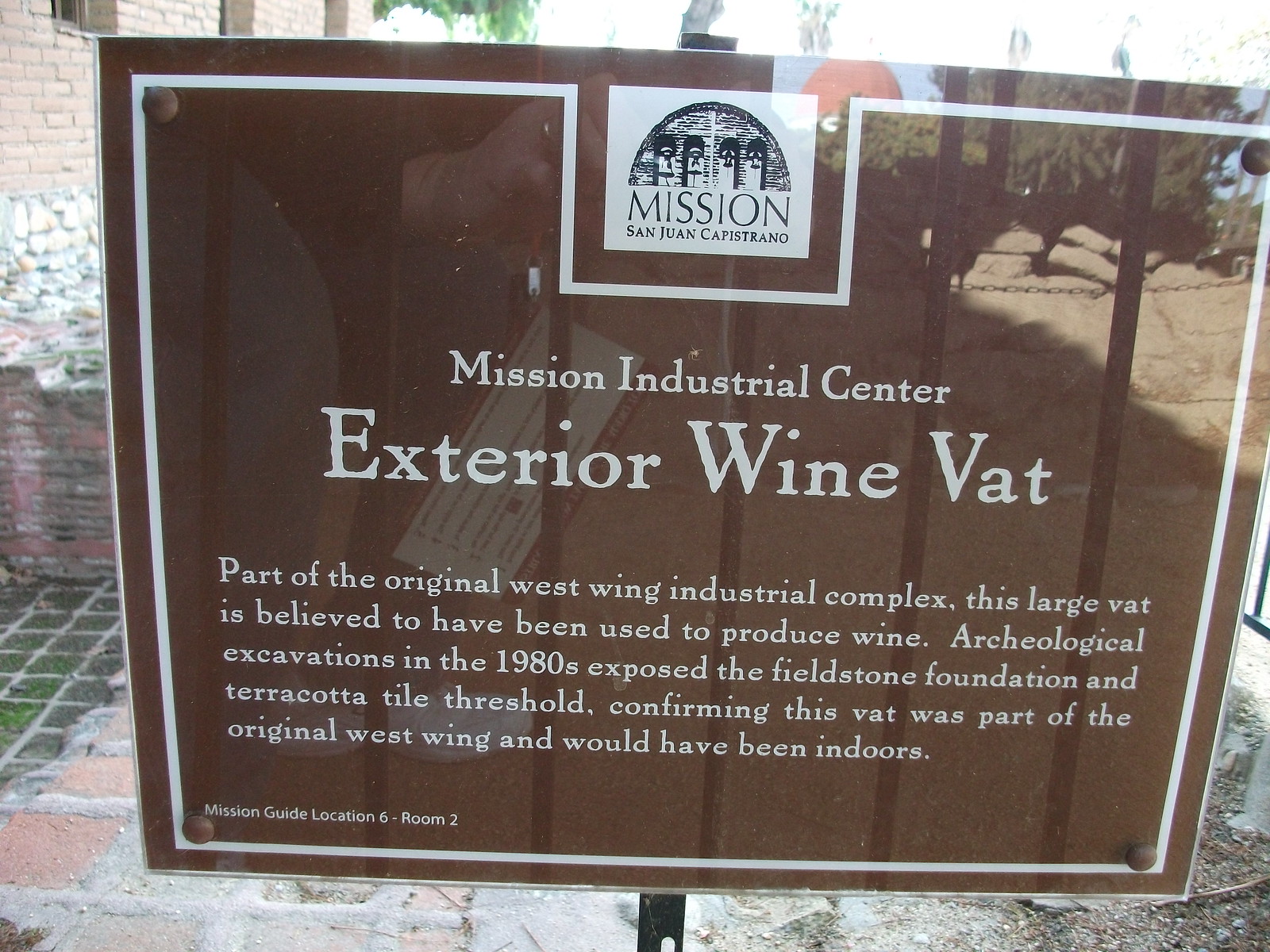The image predominantly features a reflective brown sign with a white border and white text, displayed outdoors. This sign is encased in glass, making the surface shiny with clear reflections of surrounding trees, a bench, and the ground. The sign stands upon a visible pole at the bottom middle of the image. Directly behind the sign, a brick building is noticeable, adding a textured backdrop.

At the top of the sign is the logo and name "Mission San Juan Capistrano" in black and white. Below this, slightly smaller white text reads "Mission Industrial Center," and in larger, bold white letters underneath, it states "Exterior Wine Vat." Following this is a detailed descriptive paragraph: "Part of the original West Wing Industrial Complex, this large vat is believed to have been used to produce wine. Archaeological excavations in the 1980s exposed the field stone foundation and terracotta tile threshold, confirming this vat was part of the original West Wing and would have been indoors." In the bottom left corner of the sign, it mentions "Mission Guide Location 6, Room 2." The scene appears to be taken in daylight, suggested by the bright lighting and natural reflections on the sign's surface.